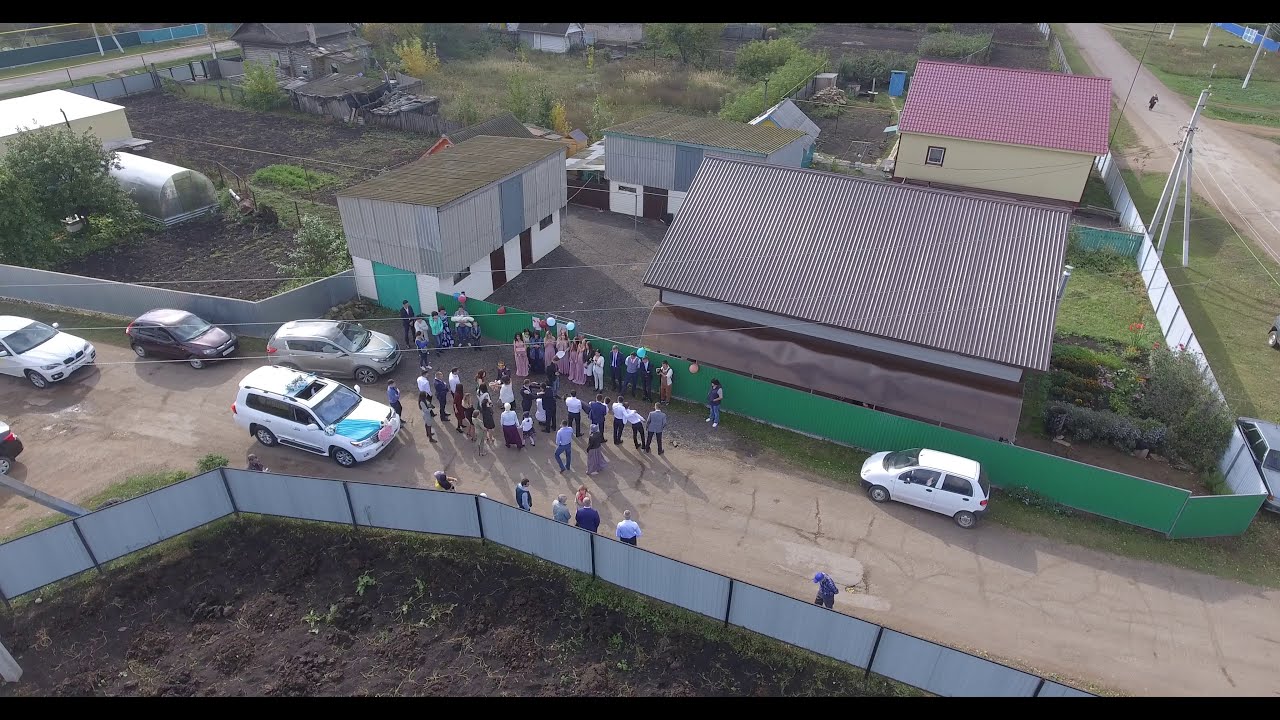This overhead shot, likely taken from a drone, captures a vibrant scene of a wedding reception in a rural area. The setting appears to be a modest agricultural community, identifiable by the metal-roofed buildings and patches of farmland. Surrounding the main event, some houses have gardens and even a greenhouse, while a dilapidated farmhouse stands in the background, reinforcing the rural character of the locale.

In the central alleyway between buildings, a large crowd has gathered for the celebration. People are mingling and dancing, with a prominent line of bridesmaids in pink dresses posing for photographs. The street is adorned with festive decorations, including balloons on fences and a white SUV festooned with a blue sash, pink and white hearts, and flowers—further indicating the joyous occasion.

The roadway is bustling with parked vehicles and attendees, forming three distinct lines along the metallic, silver, and green fence boundaries. The overall scene is a lively, communal event, rich with activity and rural charm.